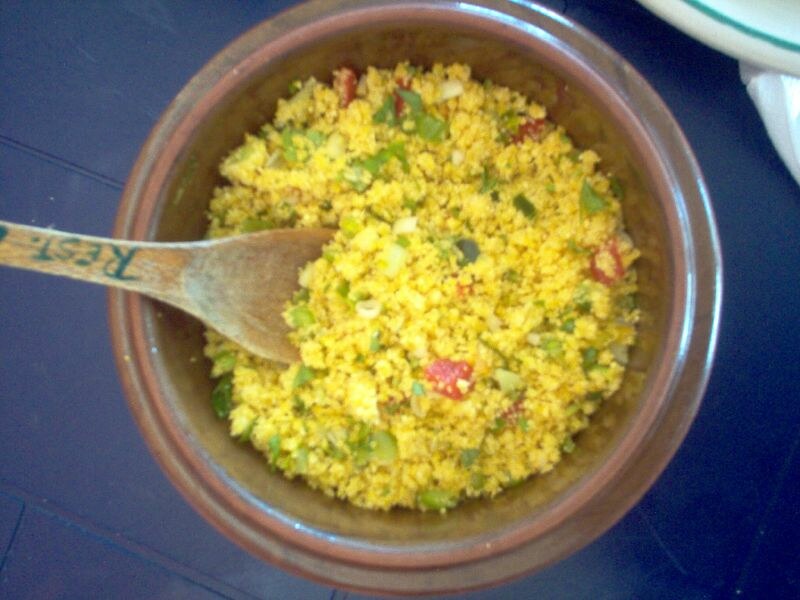In this slightly blurry photograph, a wooden bowl brimming with food sits prominently at the center of a blue table. The bowl contains what appears to be finely crumbled scrambled eggs mixed with an array of colorful vegetables, including green and red peppers, and onions. A wooden spoon, inscribed with the letters "R-E-S-T" written upside down, sticks out from the left side of the bowl. The overall color palette of the image includes various shades of brown, yellow, red, green, and a teal hue, contributing to the vibrant scene. In the upper right corner of the image, the edge of a plate, slightly cut off, is visible. The context of the setting suggests that the photo could have been taken either in a kitchen or a restaurant.